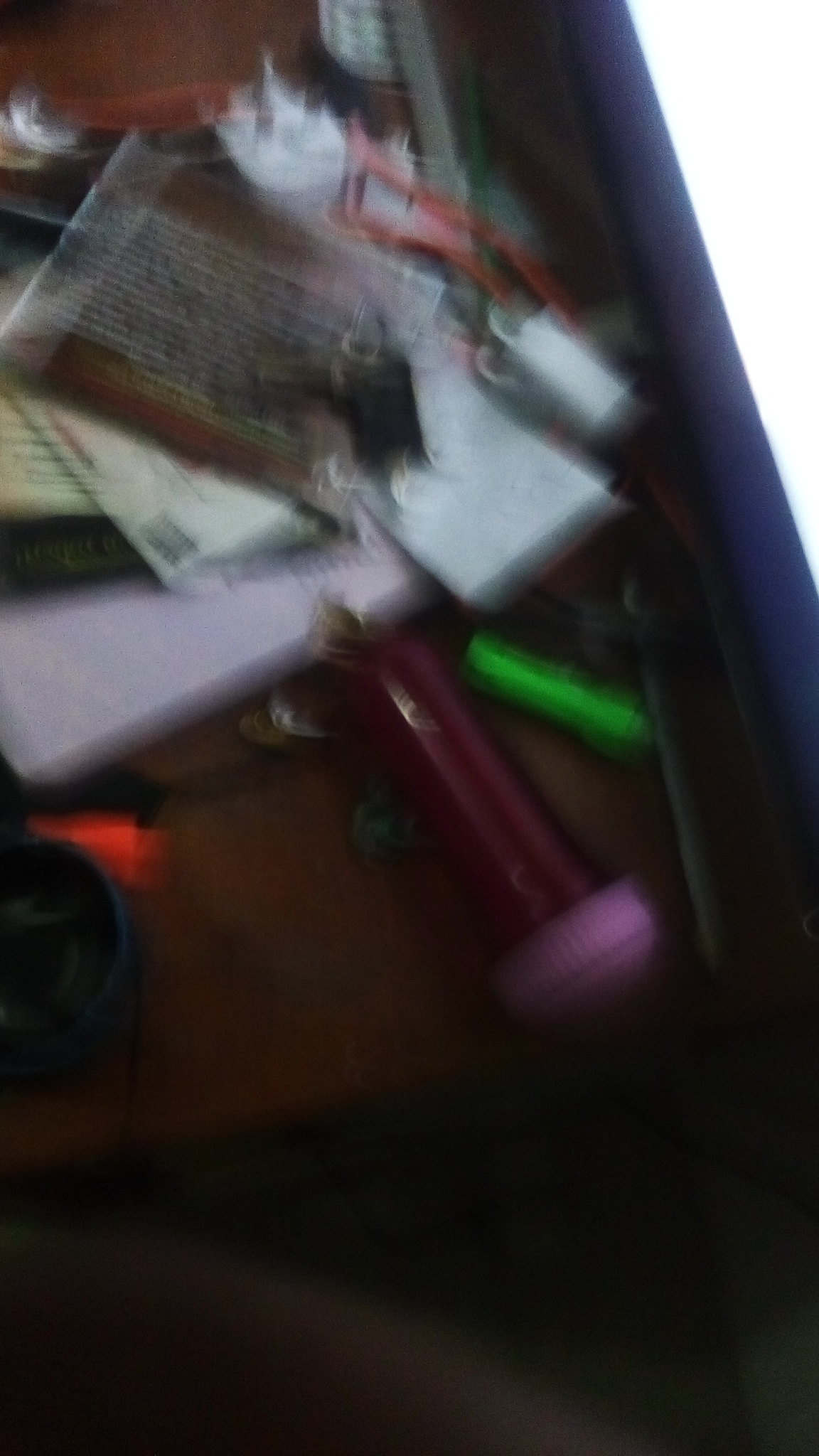In the image, a dark brown table cluttered with various items takes the spotlight, though it is captured in a somewhat blurry manner. Among the disordered collection are keys; a purplish bottle with a lighter purple cap; and an orange marker top alongside a green marker. Scattered coins, a black object in the bottom left resembling a headphone component, and a CD case are discernible amidst the chaos. An orange wire coils next to a white electrical plug with metallic prongs. On the right, a bright, blinding white light emanates from an unclear source, possibly a window or monitor. The table's edge is visible at the bottom of the image, revealing shadowy darkness below with cables snaking across the floor.